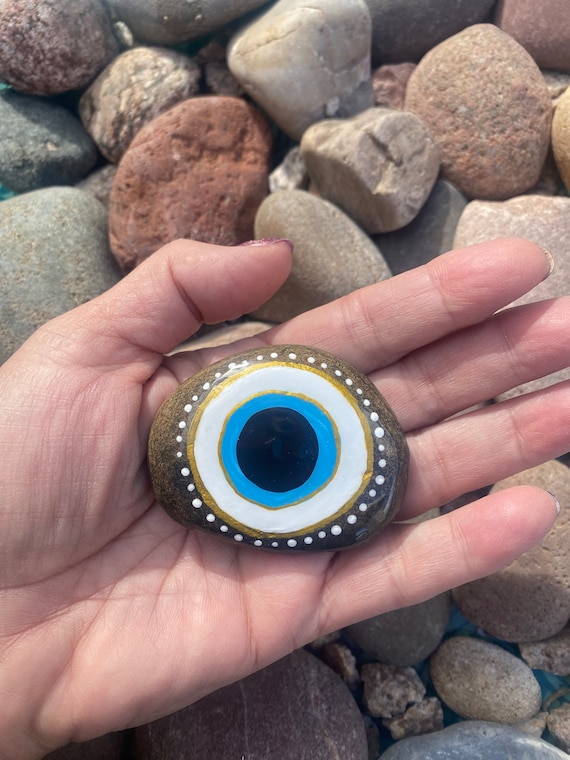This color photograph, presented in portrait orientation, features a close-up of a person’s outstretched hand entering the frame from the bottom left and middle, with the thumb pointing towards the top left. The hand, marked by visible creases in the palm and fingers, holds a smooth, elliptical brown rock intricately painted with a striking evil eye design. The center of this eye comprises a large black circle, encircled by bright turquoise, gold, white, and another gold band, respectively, all surrounded by tiny white dots. The vivid design stands out vividly against the brown stone.

Behind the hand, the background is filled with an assortment of smooth rocks in various colors. Notable among them are red, black, gray, and brown stones towards the top, with gray and brown ones towards the bottom. A hint of something blue is visible in the bottom right, contrasting with the predominantly rocky scene. This photograph, characterized by a realistic representational style, captures the detailed textures and vibrant colors of both the hand and the painted rock, set against a naturally muted rocky backdrop.